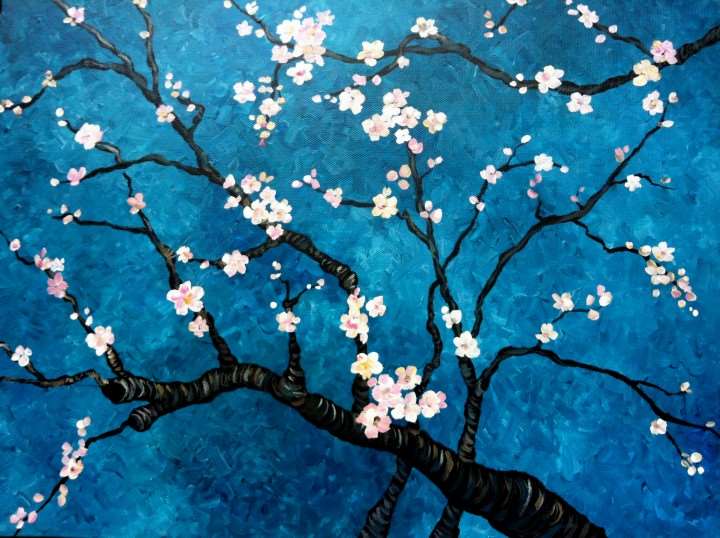The piece of art is a painting featuring a striking blue background with various shades ranging from light to dark navy, giving it depth and texture as if applied by a delicate brush. Prominently centered in the artwork is a flowering tree, reminiscent of a cherry blossom with noticeable Asian influences. The tree, depicted in shades of dark to light brown with deep blackish-blue branches, appears to be in the early stages of blooming. Its branches extend in all directions, adorned with both budding and fully bloomed flowers. The flowers are white with light pink hues and five petals each, featuring subtle yellow centers, creating a stark contrast against the deep blue backdrop. The branches are devoid of leaves, focusing solely on the vibrant, eye-catching blossoms that bring the entire composition to life.